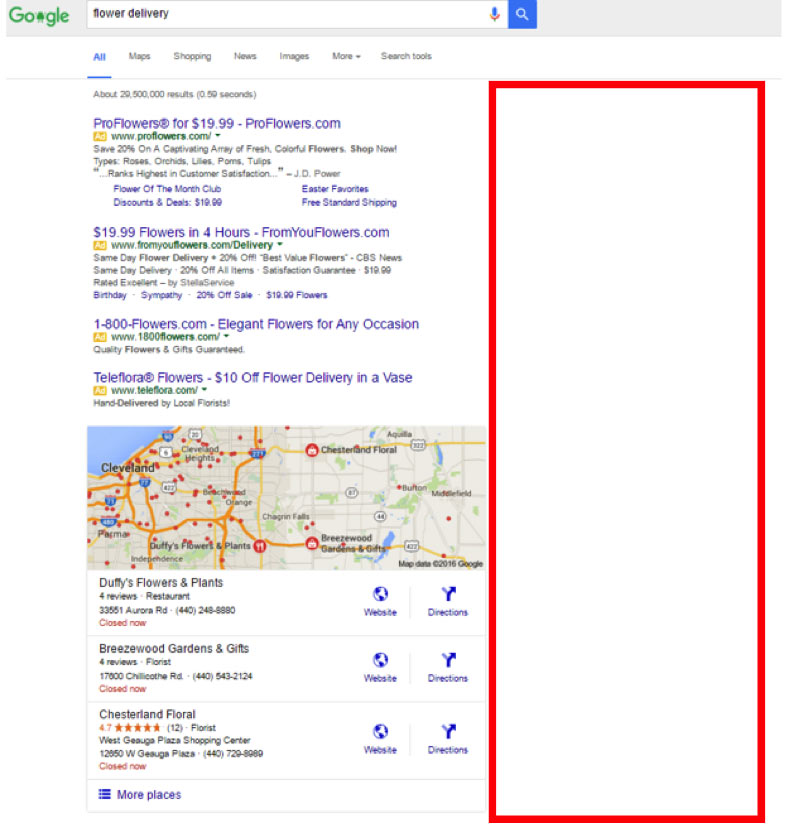The image portrays a Google search results page featuring flower delivery options. Prominently displayed in the top left is the Google logo, with a Google search box positioned at the top of the screen. The search query "flower delivery" yields several results listed from top to bottom. 

The first result is for Pro Flowers, priced at $19.99, from proflowers.com. The text highlights a 20% discount on a diverse range of fresh, colorful flowers with an invitation to shop now. Available flower types include roses, arches, lilies, pooms, and tulips. Pro Flowers is notably ranked highest in customer satisfaction by JD Power. Additional links offer options for Flower of the Month Club, discounts and deals at $19.99, Easter favorites, and free standard shipping.

The second result comes from yourflowers.com, advertising $19.99 flowers with a promise of delivery within 4 hours. The description mentions same-day flower delivery with a 20% discount on the best value flowers, endorsed by CBS News. It reiterates the satisfaction guarantee, 20% off all items, and a price point of $19.99, rated excellent by Stella Service.

The third result showcases 1800flowers.com, promoting elegant flowers suitable for any occasion, with an assurance of quality flowers and gifts. 

The fourth result is from Teleflora, which offers $10 off flower delivery in a vase, emphasizing hand delivery by local florists.

A map of Cleveland, Ohio, appears on the right side of the page, pinpointing various relevant businesses. Three florists are listed below the map: 

1. Duffley's Flowers and Plants, featuring four reviews, located at 33551 Aura Road. The contact number is 440-248-8880, with links for the website and directions.
2. Breezewood Gardens and Gifts, also with four reviews, situated at 17000 Chillicothe Road. Their phone number is 440-543-2124, alongside a website and directions links.
3. Chesterland Floral, boasting a 4.7-star rating, located at 12650 West Geauga Plaza in the West Geauga Plaza Shopping Center. Their contact number is 440-729-8989, with links to the website and directions.

At the bottom of the screen, there are additional options to view more places.